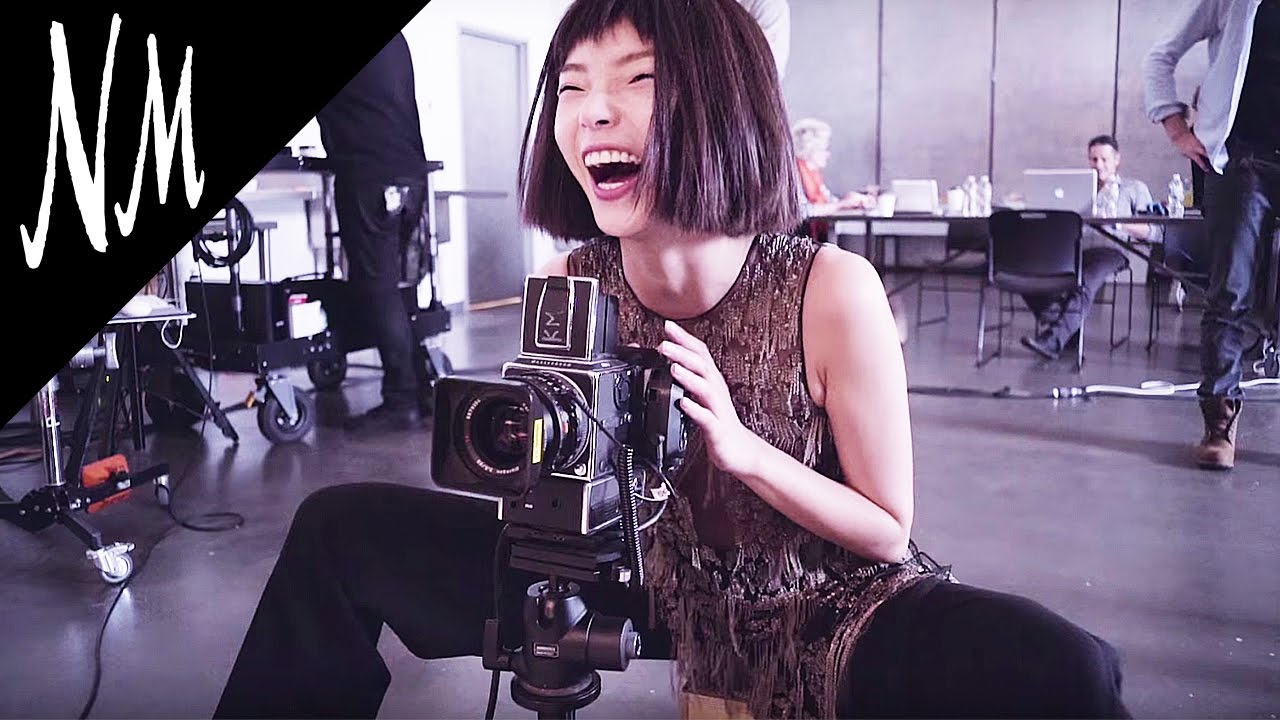In an office space, a young Asian woman sits on a very low surface near the floor, operating an old vintage camera with a large telephoto lens. She bursts into hearty laughter, her mouth wide open, eyes squinting, and legs spread wide, emphasizing her playful demeanor. Dressed in black pants and a bronze-colored tank top, her straight, neck-length hair with long bangs frames her beaming face. In the background, several people are visible: a man working on a MacBook, another man standing behind the woman, an older lady seated at a table, and a guy with equipment partially obscured by a corporate Neiman Marcus logo in the upper left-hand corner of the image. The dynamic office scene is filled with activity, adding depth and context to the woman's joyful moment.